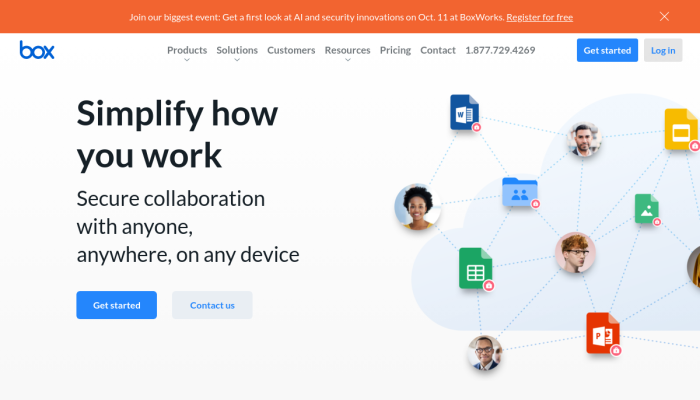Join us at BoxWorks on October 11th for an exclusive first look at groundbreaking artificial intelligence and security innovations. Register for free today and be part of our biggest event yet. A dark orange banner at the top of the page provides a clear call-to-action, with an option to close it if desired. Below the banner is the subtly bolded Box logo in lowercase letters, alongside navigational links including Products, Solutions, Customers, Resources, Pricing, Contact, Get Started, and Log In.

Central to the page is a vibrant image that depicts a diverse group of individuals— a woman, a younger man, an older man, and a black gentleman in his 30s— engaging with colorful, illustrated folders. This visual representation highlights Box's mission to simplify work and enable secure collaboration with anyone, anywhere, on any device.